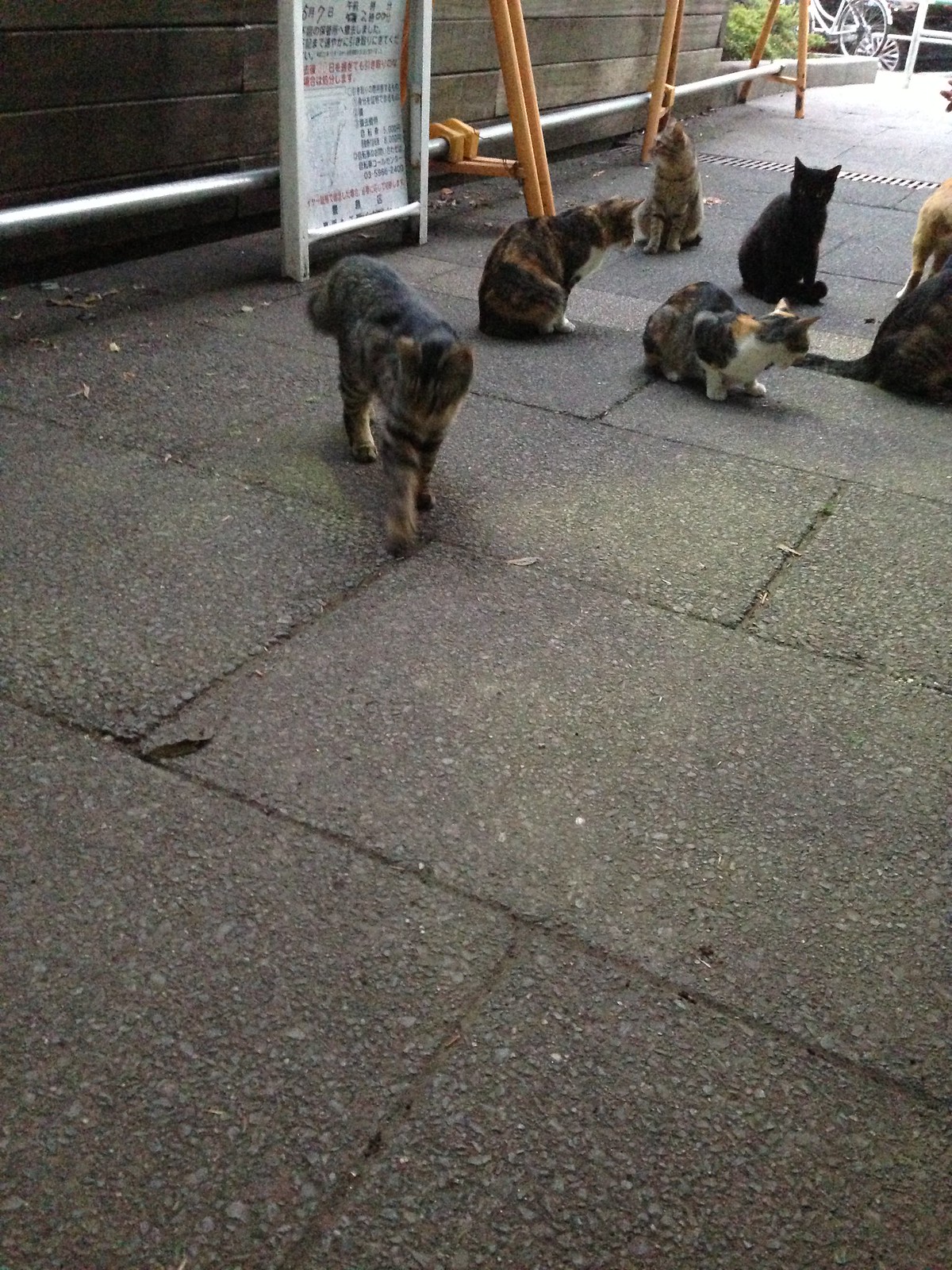The photograph captures a clean, grey pavement divided into large rectangular sections, extending from the foreground towards the back of a tunnel-like passage. The sidewalk takes up about two-thirds of the image, with the upper third showcasing a wall made of wooden planks. Along this wall are multiple pipes and a metal bar at ankle height. Near the left side of the wall, a white sign adorned with Asian characters in reds, blues, and green shades is prominently displayed. Yellow poles, possibly for bike attachment or to block vehicular access, mark the pathway. In the background, there's a lighter pavement and a grate on the floor, with part of a bike's back wheel visible.

The primary focus of the photograph lies in the seven cats scattered across the pavement. Six cats are clearly visible, while the seventh is partially cut off on the right side of the image. The cats exhibit a variety of colors: predominantly calico with their mixed patches of colors, along with one black cat positioned centrally among the calicos, and others showing shades of tabby and white. They all appear well-fed and are seated separately, some looking directly towards the camera while others gaze off into the distance. The scene, filled with a mixture of calm and watchful felines, adds a lively touch to the structured urban environment.